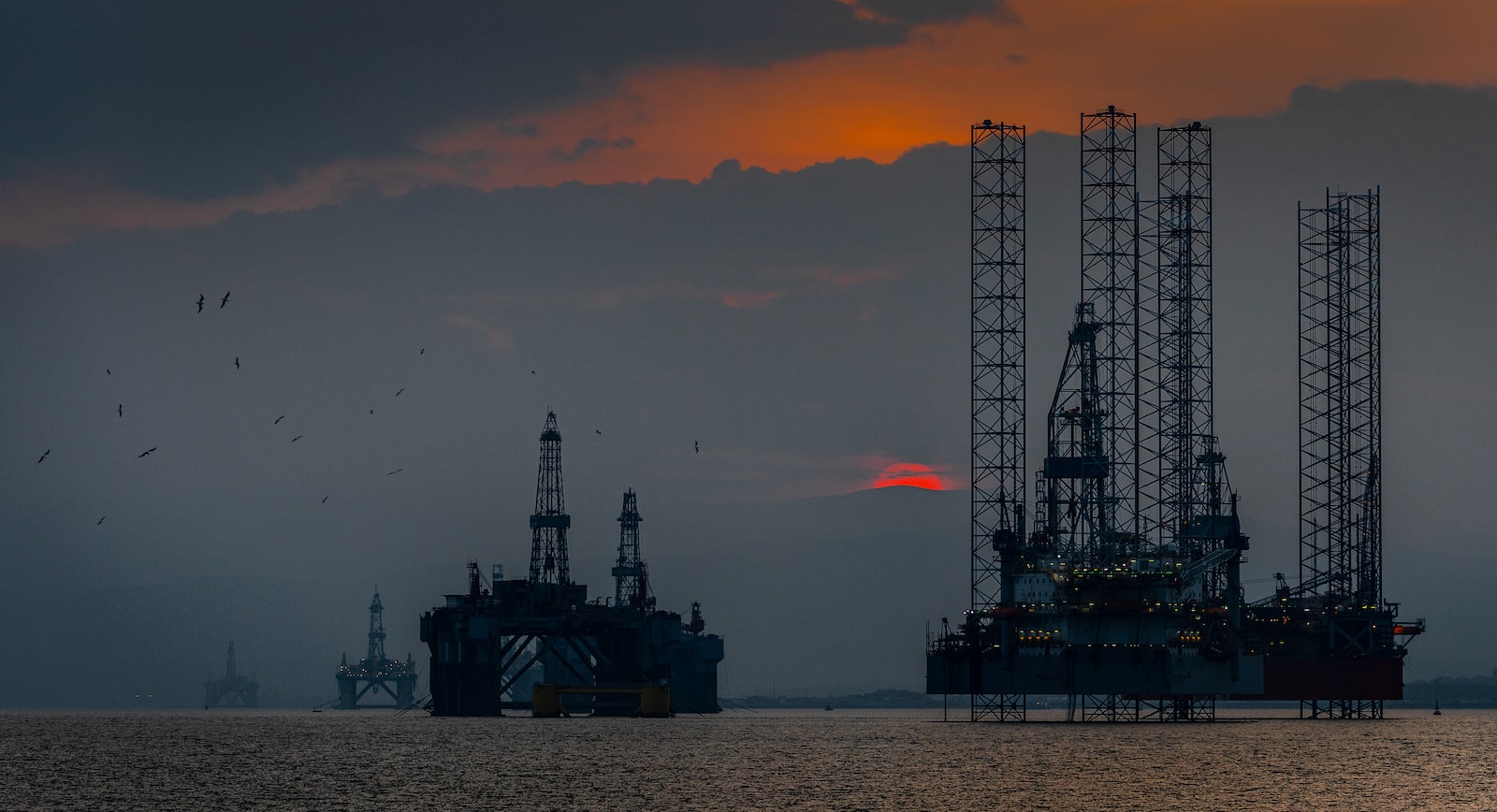The image captures a dramatic post-sunset scene on the ocean, where the last moments of the day fade into night. The upper portion of the image showcases a strikingly dark and cloud-filled sky, with a narrow strip of glowing orange near the top edge. Amidst this moody atmosphere, a deeply red, setting sun partially peeks through an opening in the overcast sky, casting its unusual dull light. 

Below this captivating sky, the ocean appears calm and almost black in color. Dominating the scene are four oil drilling platforms extending into the distance. The closest platform stands robustly on the right, featuring a large base with intricate steel girders and lattice structures that stretch upward, alongside a number of lights likely indicating human activity. To the left, additional platforms trail off into the background, decreasing in visibility and scale, with the farthest blending almost seamlessly into the dark-blue clouds. Each platform is equipped with complex metal frames, some resembling triangular structures that reach downward toward the ocean's surface. 

Overall, the image engulfs the viewer in a serene yet industrial tableau, characterized by the contrasting elements of natural beauty and mechanical prowess against a backdrop that fades steadily into night.